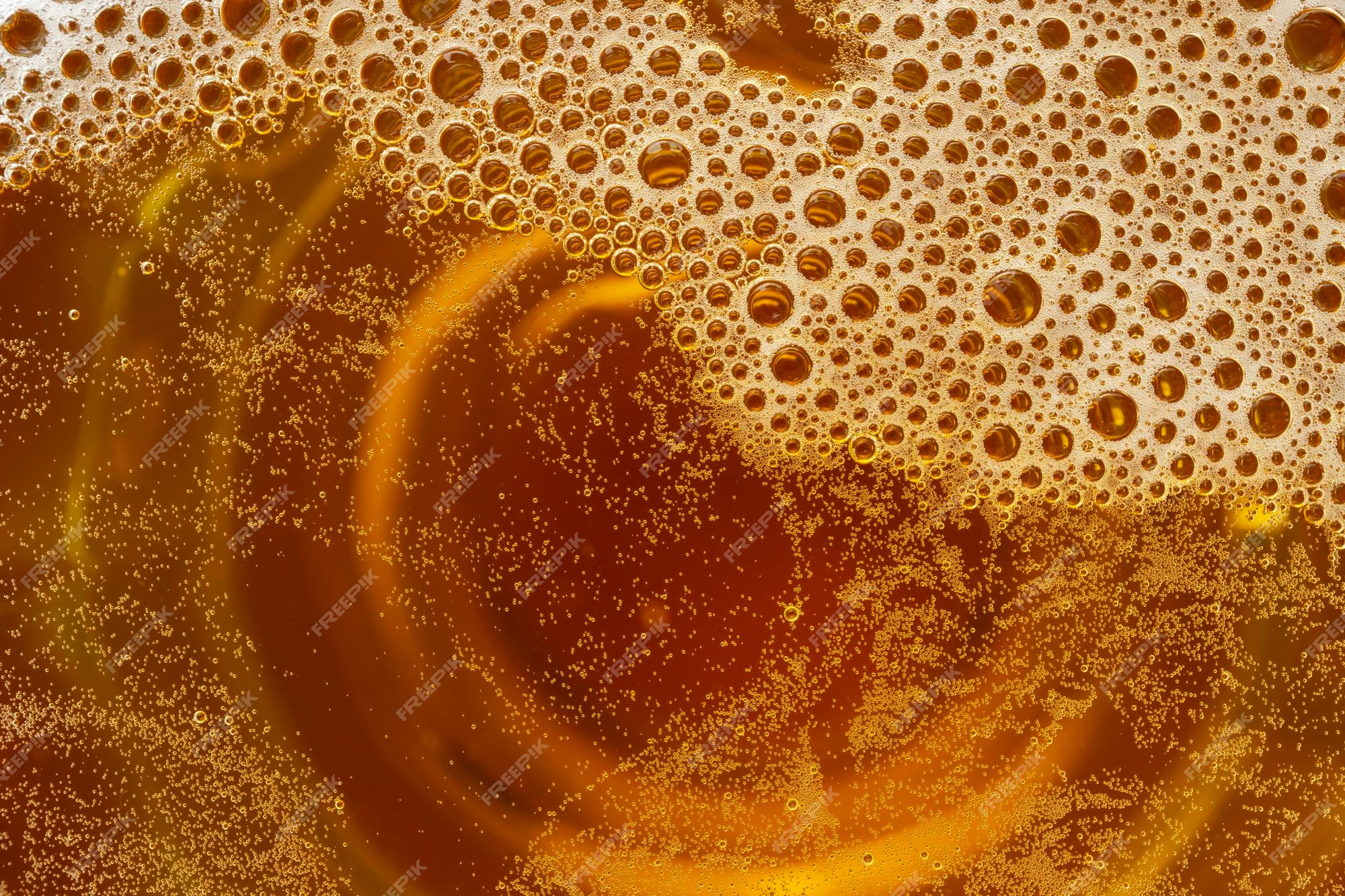The image depicts a top-down view of a glass of beer with a brownish-yellow, or deep yellow, color. The liquid is topped with a substantial layer of coarse white foam, interspersed with clear bubbles that allow a glimpse into the liquid's golden depths. Below the frothy surface, the beer features numerous bubbles rising up through the liquid. The base of the glass, visible through the liquid, has a swirling, circular pattern which might be mistaken for large, coiled noodles or the container's design. The image, marked with a watermark from "Freepik," suggests it was sourced from a free art website. Overall, the picture emphasizes the beer's rich color, the prominent frothy head, and the swirling pattern at the bottom of the glass.